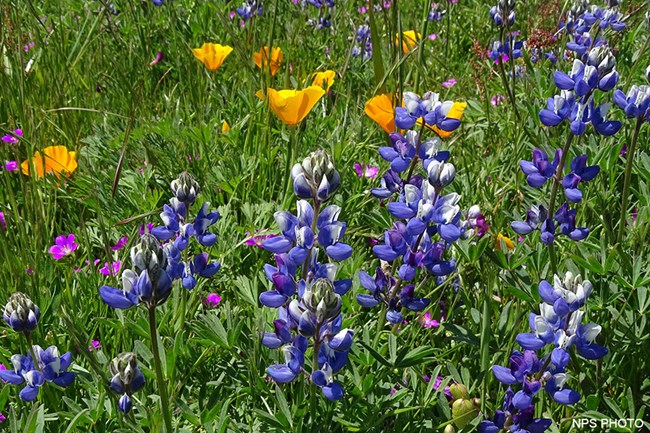The image depicts an up-close view of a vibrant field filled predominantly with bluebonnets, recognized as the state flower of Texas. The beautiful blue and white blossoms of the bluebonnets stand out, supported by lush green stems, and dominate the foreground of the photograph. Interspersed among the bluebonnets are a variety of other wildflowers, including a scattering of shorter purple flowers with white centers, and tall golden-yellow flowers, possibly buttercups. The scene also showcases an array of smaller, light pink fuchsia and lilac-colored blooms, lending a rich tapestry of colors. The entire scene, bathed in natural light, suggests an outdoor, wooded, or meadow-like setting. In the bottom right corner of the image, the text "NPS Photo" is prominently displayed in white lettering.